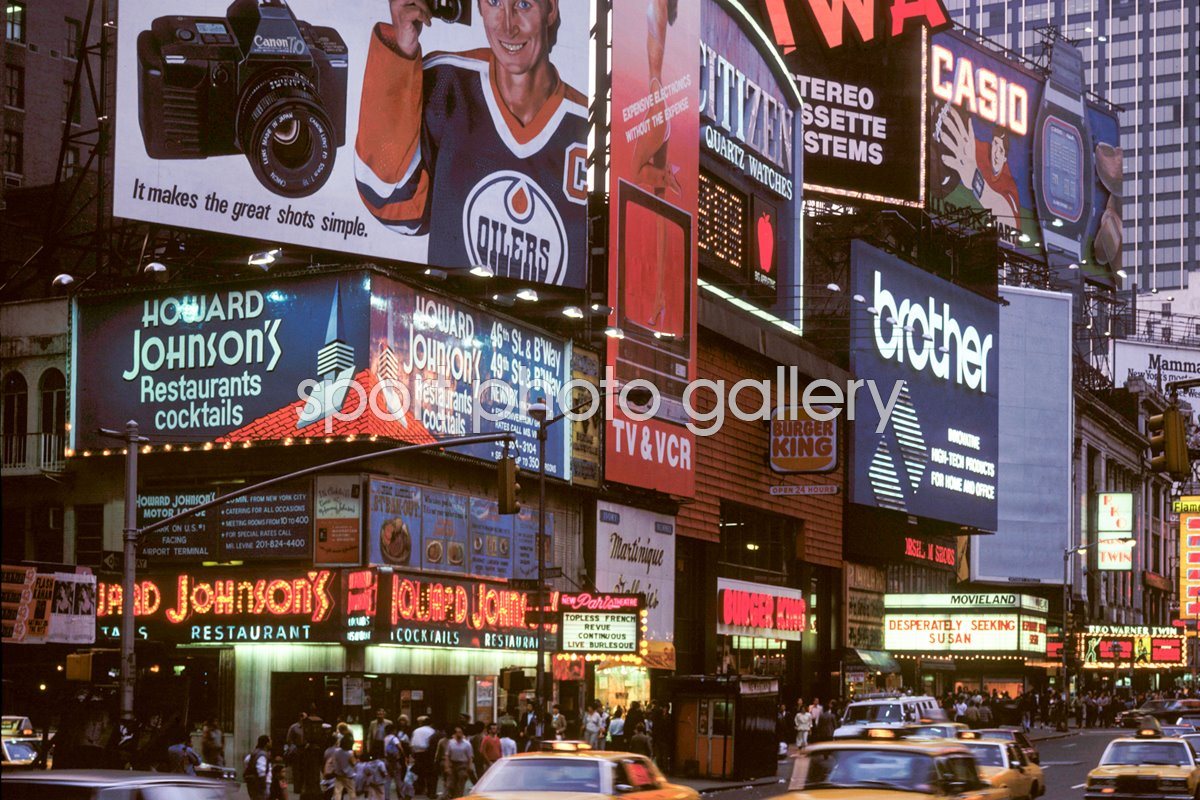This photograph, likely from the 1980s, captures a busy street scene in New York City's Times Square at dusk. The street is bustling with energy as numerous yellow taxi cabs navigate the roadway, their lights glowing, while throngs of pedestrians fill the sidewalks and crosswalks. The storefronts and billboards are vibrant with advertisements, casting colorful lights across the scene. Notable signs include a Howard Johnson's Cocktails Restaurant with a prominent neon sign, an advertisement for a Canon camera featuring a Texas Oilers player, and a Casio sign depicting someone playing a keyboard. Other signs highlight Burger King, Brother office products, and a marquee for the movie "Desperately Seeking Susan," which firmly places the image in a bygone era. The lively mix of reds, blues, blacks, yellows, and whites in the advertisements, paired with older car models including the yellow cabs, reinforce the photograph’s nostalgic atmosphere. A watermark reading "Sport Photo Gallery" subtly overlays the image, adding to the historical documentation of this vivid urban tableau.